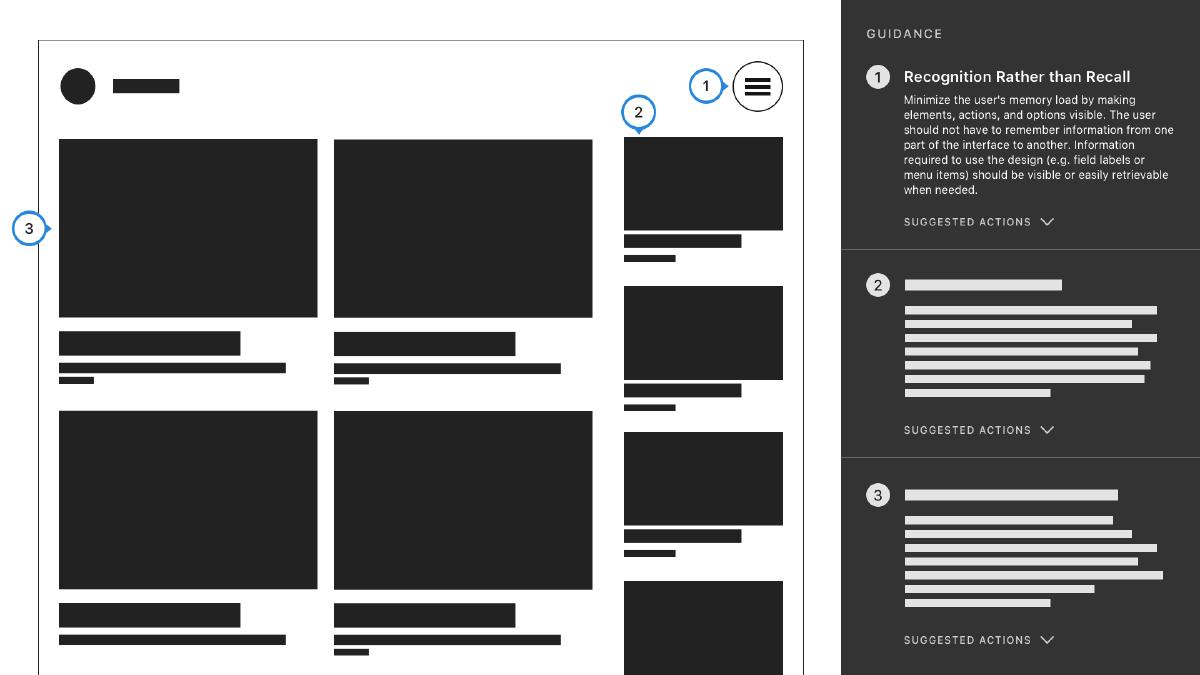A person appears to be giving a presentation, utilizing a display divided into distinct sections. In the top left corner, there is a large white box with a solid black circle. Adjacent to this box, towards the right, there is an elongated, narrow rectangle. Directly below this, a substantial black box features three circular markers on its left side. An identical black box is positioned to the right of this one. 

Below each of these larger black boxes, there are two sets of smaller, horizontal boxes arranged vertically, mirroring one another. This pattern is repeated, resulting in a grid-like formation of identical black and grey boxes.

On the top right side, there are three parallel horizontal lines enclosed within a circle; extending from this setup is a line leading diagonally downwards to a smaller rectangle marked with the number "2." Below this, arranged vertically, there are four larger black boxes with horizontal boxes beneath each one, maintaining a consistent styling.

To the far right, there is a vertical black box labeled "Guidance." It contains text reading "1. Recognition rather than recall: Minimize the user's memory load by making elements, actions, and options visible." Below this section, indicated by a dividing line, there are spaces marked as "Suggested actions" filled with white-out-like strips. A similar structure is designated for "2" and "3," each featuring additional "Suggested actions" sections filled with further strips resembling white-out blocks.